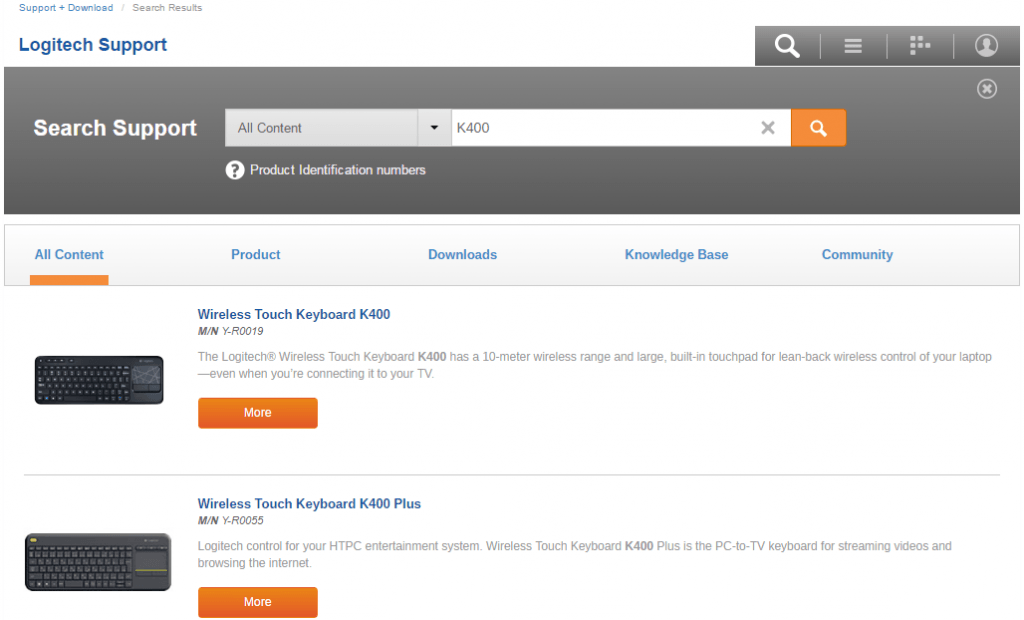**Detailed Caption for Screenshot of Logitech Support Webpage**

The image is a screenshot of the Logitech Support webpage. At the top of the page, the header reads "Logitech Support" with the text specifically spelled out as "L-O-G-I-T-E-C-H Support." Just above this label, there is additional navigation information displayed: "Support + Download / Search Results" followed by "Logitech Support."

On the upper right-hand corner of the screen, several interactive elements are present: a search button, a three-lined menu icon for additional options, a Logitech logo, and a blank profile picture icon indicating user options.

Below the header, a large gray bar spans the width of the page. In white text, the bar features the words "Search Support, All Content," next to a search input box containing the query "K400." An orange search button is positioned beside the input box.

Further down, the text "Product Identification Numbers" appears in white, still positioned on the gray bar. Below this, the page contains navigation tabs: "All Content," "Product," "Downloads," "Knowledge Base," and "Community." The "All Content" tab is currently selected, indicated by an orange underline beneath it.

The main content of the webpage lists two products. 

1. **Product Listing 1**:
   - **Image**: On the left, a black keyboard is shown.
   - **Name and Model**: "Wireless Touch Keyboard K400," with the product identification number "N/N-Y-R-0019."
   - **Description**: "The Logitech Wireless Keyboard K400 has a 10-meter wireless range and a larger built-in touchpad for lean-back wireless control of your laptop, even when you're connecting it to your TV."
   - **Call to Action**: An orange button labeled "More."

2. **Product Listing 2**:
   - **Image**: A gray keyboard with a large touchpad is shown.
   - **Name and Model**: "Wireless Touch Keyboard K400 Plus," with the product identification number "N/N-Y-R-0055."
   - **Description**: "Logitech Control for your HTPC Entertainment System. Wireless Touch Keyboard K400 Plus is the PC-to-TV keyboard for streaming videos and browsing the internet."
   - **Call to Action**: An orange button labeled "More."

This structured layout makes it clear and easy to navigate through Logitech's support and product information for the K400 and K400 Plus wireless keyboards.